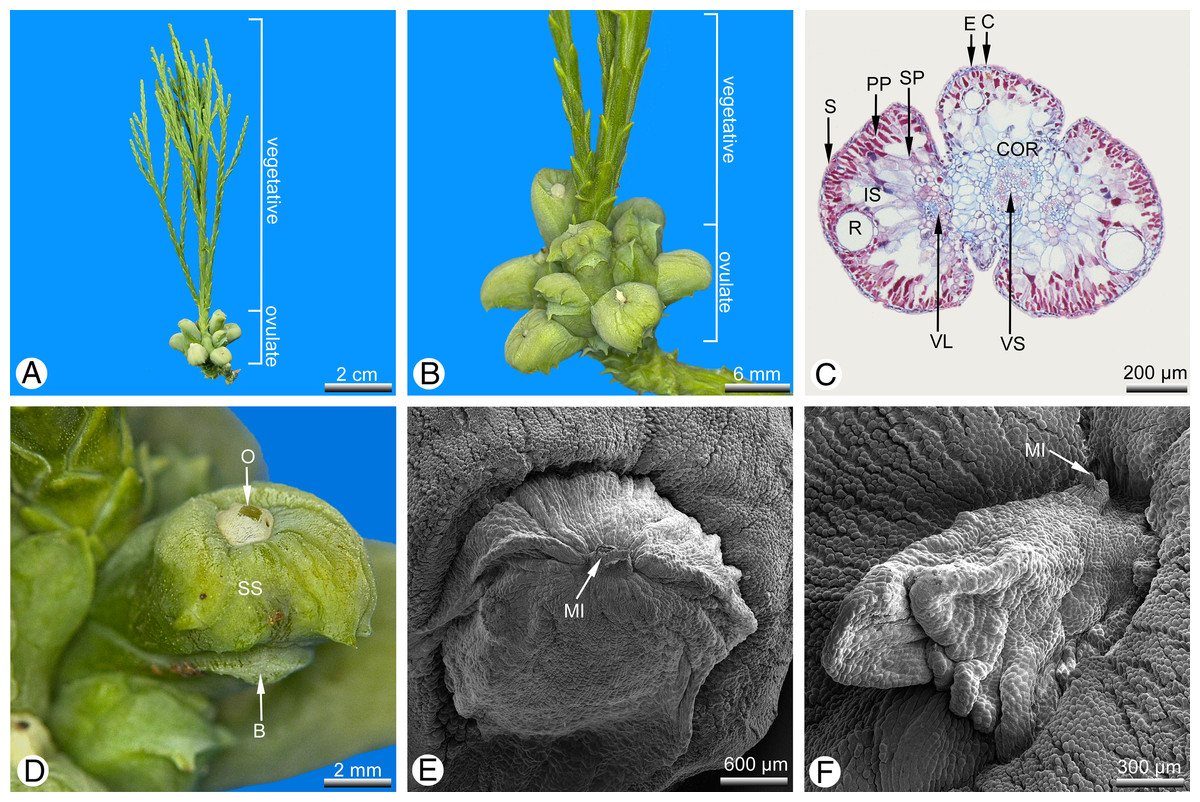The image consists of six detailed, close-up biological images, possibly of a plant, organized in two rows of three. Each image is labeled from A to F with black text inside a white circle. The labels A, B, and D are in full color, while C is partially colored, and E and F are black and white.

- **Image A** (top left) is a full-color photograph showing the entire plant with distinct sections: the "vegetative" part comprising the leaves and stalks at the top, and the "ovulate" part showing a cluster of fruit at the bottom. It includes a scale bar indicating 2 centimeters.
  
- **Image B** (top middle) provides a close-up view of the fruit cluster and part of the stem. This image is also in color and comes with a scale bar indicating 6 millimeters.
  
- **Image C** (top right) is a color-enhanced cross-section of the plant, displaying internal structures in red and blue. It is marked with a scale of 200 micrometers (200 µm) and various labeled sections.
  
- **Image D** (bottom left) features an extreme close-up of one of the fruiting bodies in full color, with specific parts labeled "B" (bottom), "O" (top), and "SS" (middle). The image includes a scale bar showing 2 millimeters.
  
- **Images E and F** (bottom middle and bottom right) are black and white electron microscope images, providing a highly magnified view of the plant's microstructures. Image E is marked with a scale of 600 micrometers (600 µm) and labels the area "MI," while Image F shows a different part, also labeled "MI," with a scale of 300 micrometers (300 µm).

Each image is precisely annotated with scale bars to give a sense of magnification, illustrating the plant from an entire structure to microscopic details.